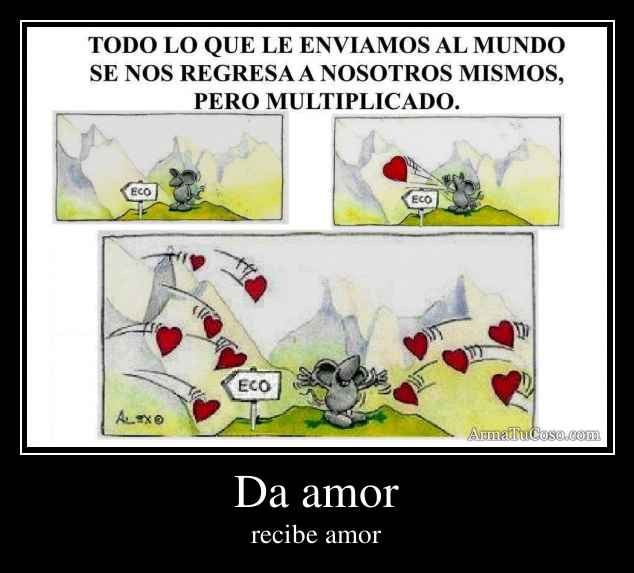The image is an animated comic strip with a Spanish title that reads "Todo lo que le enviamos al mundo se nos regresa a nosotros mismos, pero multiplicado." At the bottom, it has the phrase "Da Amor, Recibe Amor," which translates to "Give love, receive love." The poster is framed in black, featuring a white rectangle in the center divided into three horizontal panels, all depicting a little cartoon mouse. In the first panel, the mouse stands still with the word "ECO" and an arrow pointing left. In the second panel, the mouse throws his heart out into the world. In the third and largest panel at the bottom, the mouse is atop a mountain, receiving multiple hearts back as he throws more hearts into the valley. The entire scene is set against a backdrop of a mountain range and uses colors like red, lime green, olive green, gray, black, and white. The overall style of the image is reminiscent of a comic strip or meme, and it conveys the message that the love you give out returns to you multiplied.